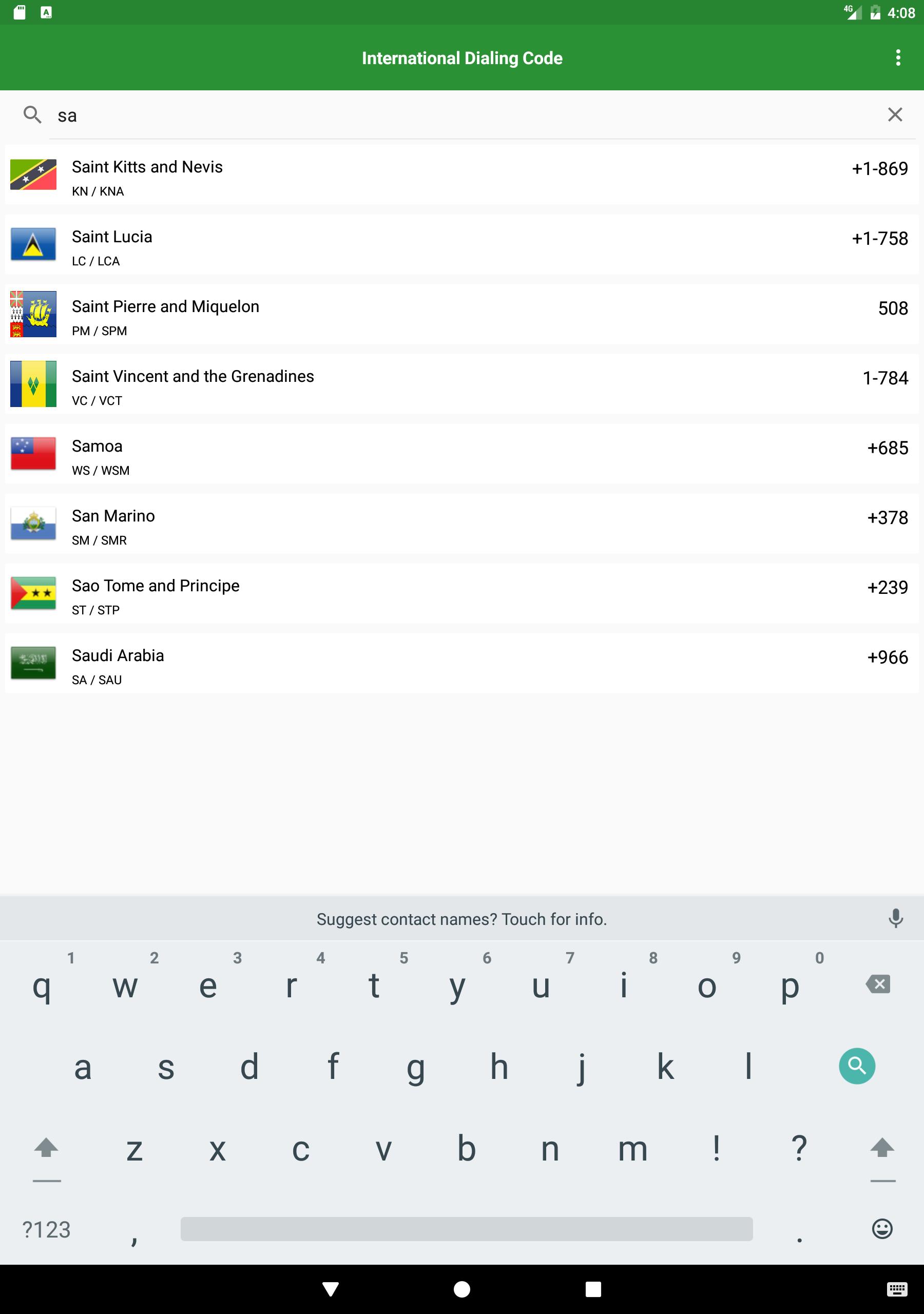The image features a white background with several elements arranged across it. At the top, there is a green rectangle, flanked by two small white boxes on the left. Below, the number four appears next to the label "International Dialing Code," accompanied by an ellipsis (...). 

Underneath, a magnifying glass icon is placed, followed by a number that appears blurred. On the right side of this section, an 'X' symbol is visible. 

The central portion lists various international dialing codes:
- St. Kitts and Nevis: +1 869
- St. Lucia: +1 758
- St. Pierre and Miquelon: +508
- St. Vincent and the Grenadines: +1 784
- Samoa: +685
- San Marino: +378
- Sao Tome and Principe: +239
- Saudi Arabia: +966

At the bottom of the image is a light blue keyboard. Above the keyboard, there is a text indicating "Suggest contact names" with a question mark and "Touch for info." 

On the right-hand side of the keyboard, a blue circle contains a magnifying glass icon, accompanied by an 'X' and a square. Further details include a microphone icon at the top, an upwards arrow, and a smiley face icon at the bottom. On the left side of the keyboard, there is another upwards arrow along with a key labeled "?123."

At the very bottom, there is a black bar featuring a triangle, circle, and square, alongside another small square icon on the right side.